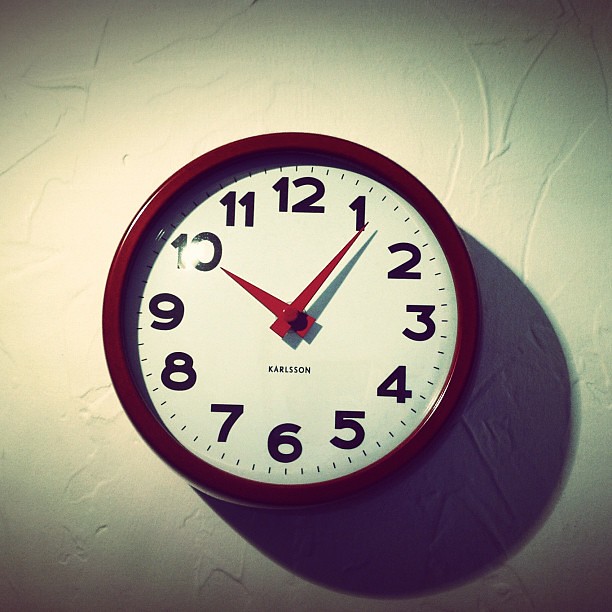The image features a Carlson clock mounted on a pristine white wall. The clock casts a pronounced shadow towards the bottom right of the image, highlighting the stark contrast created by the lighting. The clock's face is adorned with large, bold black numbers, making it easy to read from a distance. The minute and hour hands are bright red, simple, and sleek, ending in sharp points. The time displayed is 10:06, though it is unclear whether it is a.m. or p.m. The clock has a classic design often seen in institutions like police stations or schools, evoking a sense of familiarity. The maroonish-red outline of the clock adds a distinctive touch, making it stand out on the wall.